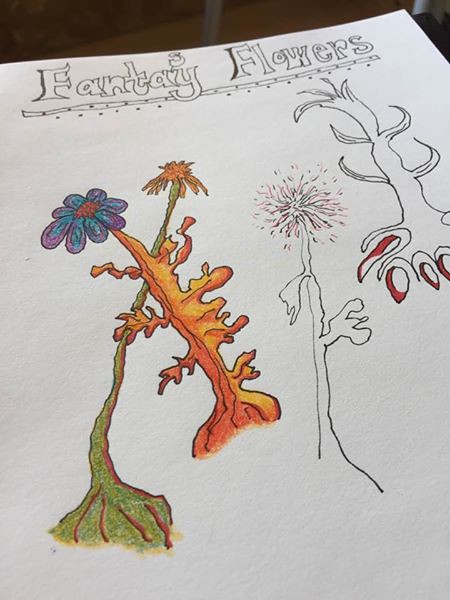This photograph captures a hand-drawn illustration on a sheet of paper titled "Fantasy Flowers." The drawing features four distinct types of fictitious flowers, each characterized by their unique and whimsical designs. The title "Fantasy Flowers" appears prominently at the top of the page, although the artist initially misspelled "Fantasy" and had to add the missing "S" afterward, resulting in an awkward visual correction that stands out. The flowers themselves are vibrant and diverse in color, showcasing hues from green and blue to orange, with these colors vividly applied to both the petals and stems of the plants. This imaginative artwork exudes creativity and a sense of otherworldly beauty.